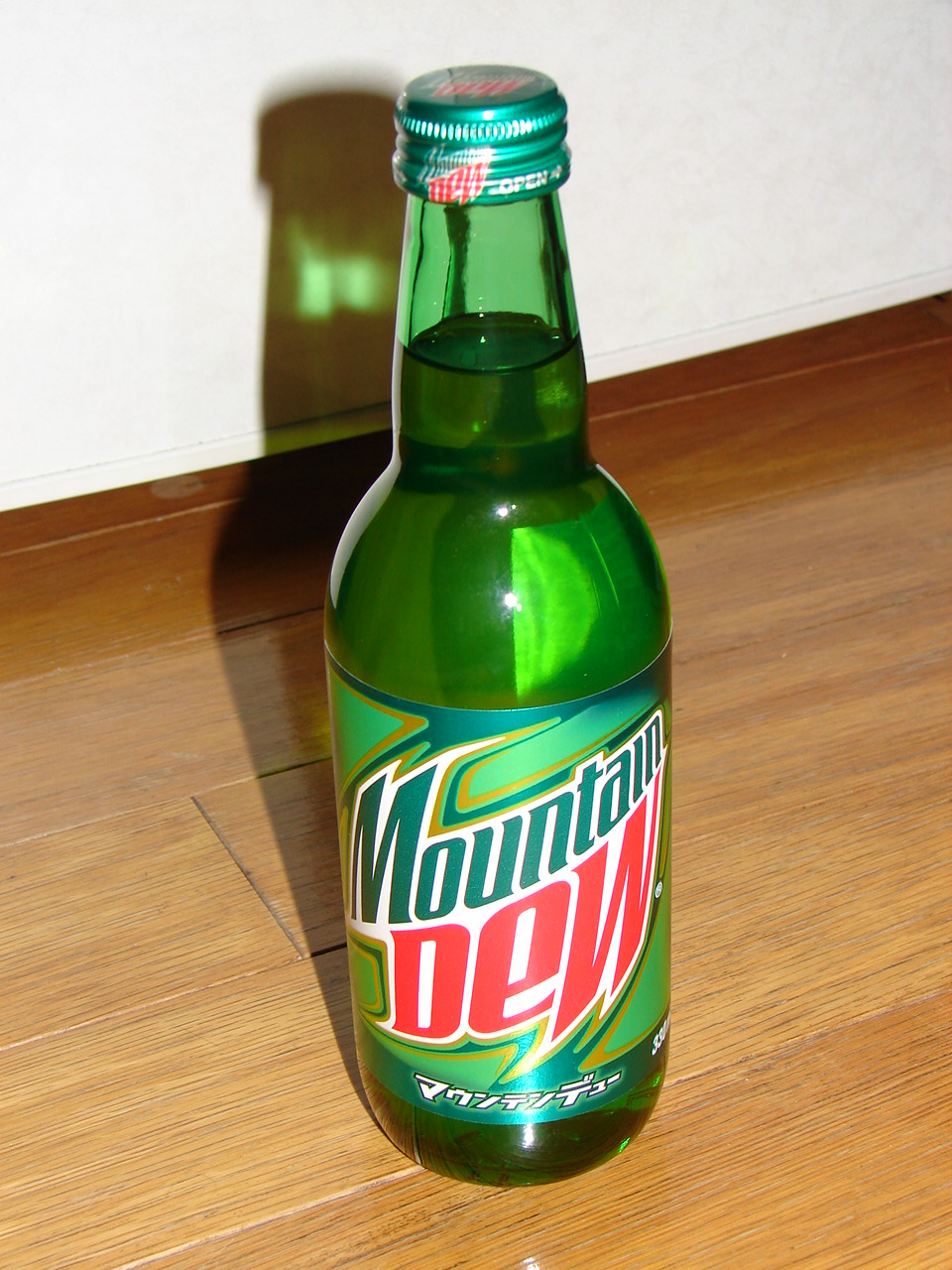A close-up photograph showcases a striking glass bottle of Mountain Dew, securely placed on a light-colored, possibly golden-hued, hardwood floor. The backdrop features a pristine white wall, complementing the overall composition. The bottle itself is predominantly green, cylindrical at the base but tapering towards the top where it meets a screw-on cap, which is a different shade of green. The liquid inside appears green through the tinted glass. The reflected light creates a prominent white shine on the bottle’s front center. The labelling features a green background with the text "Mountain Dew" prominently displayed; "Mountain" is written in dark teal and "Dew" in dark pink. Some additional text in another language is visible beneath the main label, adding an international flavor to the presentation.